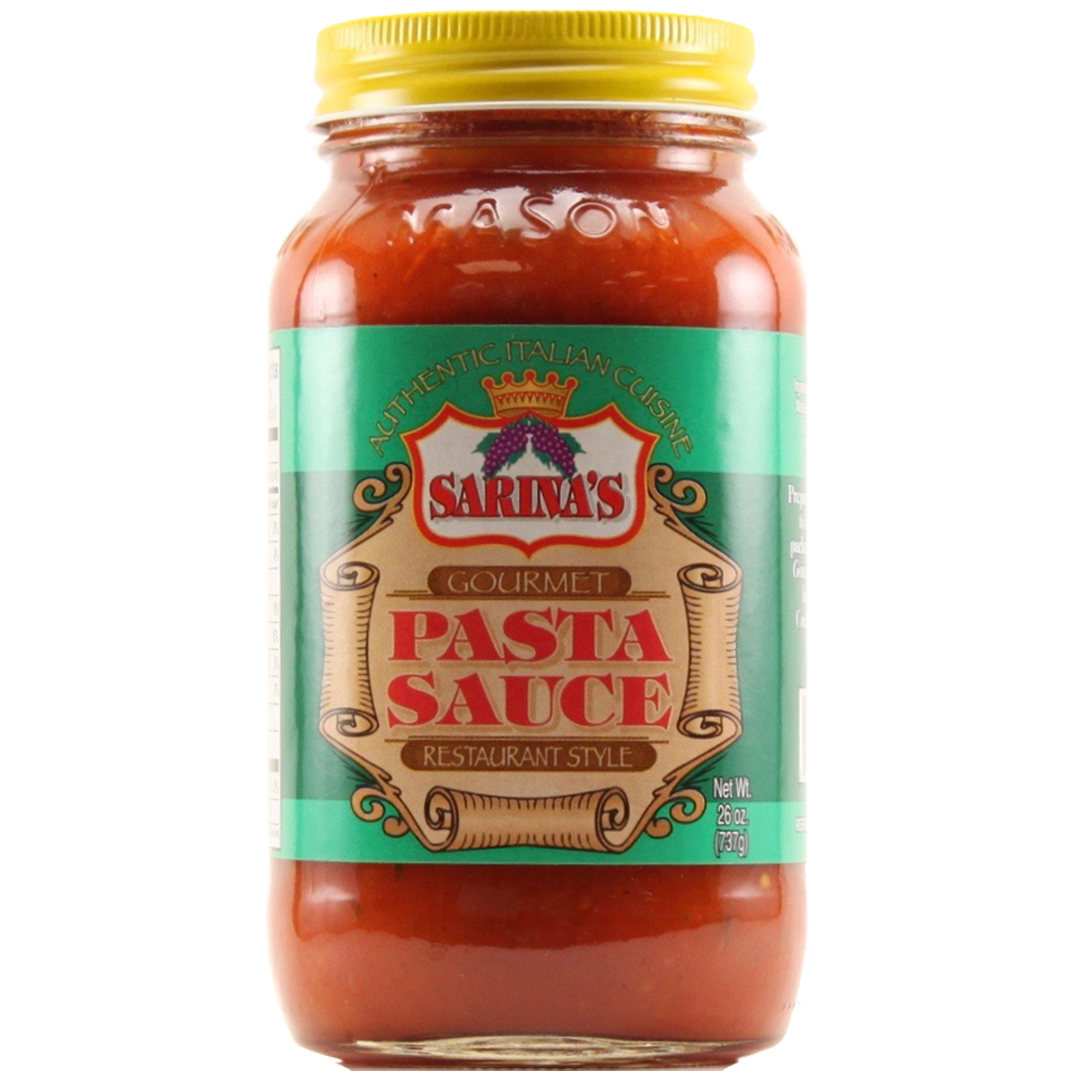This detailed photograph showcases a glass mason jar filled with vibrant red tomato pasta sauce, complete with visible herbs and seasonings. The jar is distinguished by the word "mason" raised on the glass at the top, signifying its iconic design. Topping the jar is a yellow tin screw cap. The focal point is the intricately designed label wrapped around the jar's middle. The label features a light green border with a dark green center. At the top, in yellow font, the label reads "Authentic Italian Cuisine." Below this, on an artistically-rendered scroll of light brown parchment, it states "Serena's Gourmet Pasta Sauce, Restaurant Style" in a mixture of elegant fonts. Adding to the authenticity, a golden crown and bunches of purple grapes adorn the label, enhancing the artisanal feel of the product.